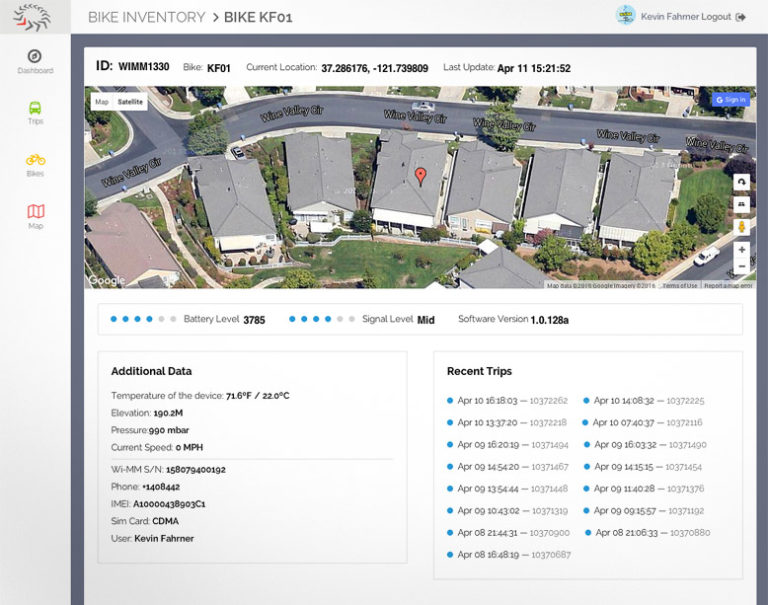The image features a detailed and complex interface, primarily themed in various shades of gray and blue. In the upper left corner, there's a composition of two gray rectangles, one slightly darker than the other. Below these, a circular arrangement of small gray shapes is displayed, with one shape distinctly marked in red. Adjacent to this circle, the text reads "Bike Inventory" with an arrow pointing to the right, leading to the label "Bike KF01".

To the right, a blue circle encloses a picture featuring green elements, accompanied by indecipherable text and an unclear symbol beside it. On the left side of the interface, a circle containing an arrow is labeled with unreadable text beneath it. Nearby, green, yellow, and map-like elements each have indistinct annotations.

Surrounding the main content is a border made up of a blue-gray line, outlining the left side, top, and right side of the image. Inside this border is a white rectangle labeled "ID," followed by a combination of letters, numbers, and gray text, with subsequent gray and black numbers, as well as a date and time stamp, appearing adjacent to what seems to be a map.

At the top, a small white rectangle contains unspecified words, with several white squares featuring unrecognizable symbols aligned along the right side. Additionally, another white rectangle is present, along with clusters of blue and gray dots interspersed with words. There are two sequences of four blue dots and two gray dots, each sequence accompanied by text.

Below, the section labeled "Additional Data" contains multiple words and numbers, succeeded by a "Recent Trips" area. This section includes several blue dots in two rows, each followed by words resembling dates.